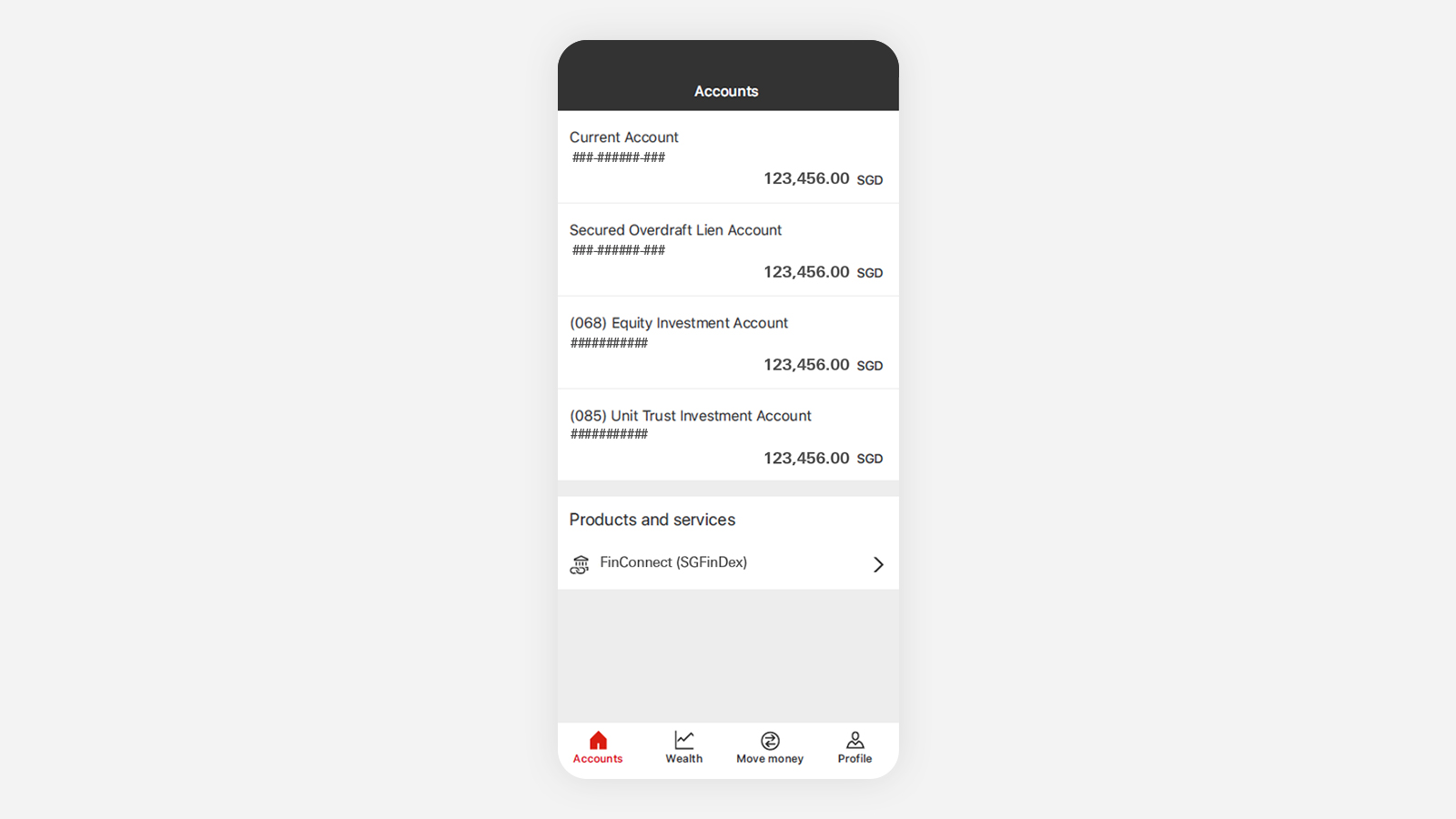**Screenshot of Mobile App Displaying Various Financial Accounts and Services**

The screenshot captures a mobile banking application interface with a dark background. At the top middle, the word "Accounts" is displayed prominently in white font. Below it, several account details are structured as follows:

1. **Current Account**: The account number is obscured with pound signs (####) and shows a balance of **123,456 Singaporean dollars**.
2. **Secured Overdraft Loan Account**: Displays a balance of **123,456 Singaporean dollars**.
3. **Equity Investment Account**: Listed as "closed" within parentheses, identified with the number **068**, and a balance of **123,456 Singaporean dollars**.
4. **Unit Trust Investment Account**: Also "closed" within parentheses, marked with the number **085**, and a balance of **123,456 Singaporean dollars**.

Beneath these account summaries, the section labeled "Products and Services" includes "FinConnect" and "Singapore Findex" with a right-facing arrow indicating further options. 

At the bottom of the screen, the navigation menu includes the following items: "Accounts", "Wealth", "Move Money", and "Profile", with "Accounts" highlighted in red, suggesting it is the currently active section.

The primary text for the account summaries is in black font on a white background, with light gray accents used for separation between account sections.

This detailed view provides an organized snapshot of various financial accounts and services accessible through the mobile app.